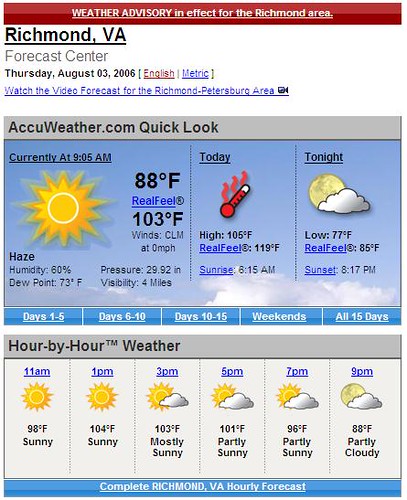Screenshot from AccuWeather.com showcasing the weather forecast for Richmond, Virginia. 

At the top of the image, there's a prominent weather advisory in white text on a red background, alerting viewers to significant conditions in the Richmond area. Below it, the location "Richmond, Virginia" is clearly displayed, followed by the "Forecast Center" in gray text. The date is specified as "Thursday, August 3rd, 2006," with options to toggle between English and Metric units. There's also a link inviting users to "Watch the video forecast for the Richmond-Petersburg area."

A detailed table shows the current weather conditions: a temperature of 88°F feels like 103°F due to 60% humidity and a dew point of 73°F. Winds are calm at 0 mph, atmospheric pressure is at 29.92 inches, and visibility is reduced to 4 miles. The high for the day is projected to be an intense 105°F, feeling like a scorching 119°F, with sunrise at 8:15 AM. The night will bring a low of 77°F, feeling like 85°F, with sunset at 8:17 PM.

Additional navigation options include tabs for "Days 1-5," "Days 6-10," "Days 10-15," "Weekends," and "All 15 Days." 

An hourly forecast is provided, indicating temperatures will peak at 104°F at 1 PM, with subsequent temperatures of 103°F at 3 PM, 101°F at 5 PM, 96°F at 7 PM, and cooling slightly to 88°F by 9 PM. 

At the bottom, a blue background with white text reads "Complete Richmond VA hourly forecast." The top section features various images, including a blazing sun, a thermometer symbolizing extreme heat, and a moon, enhancing the visual appeal and conveying weather conditions effectively.